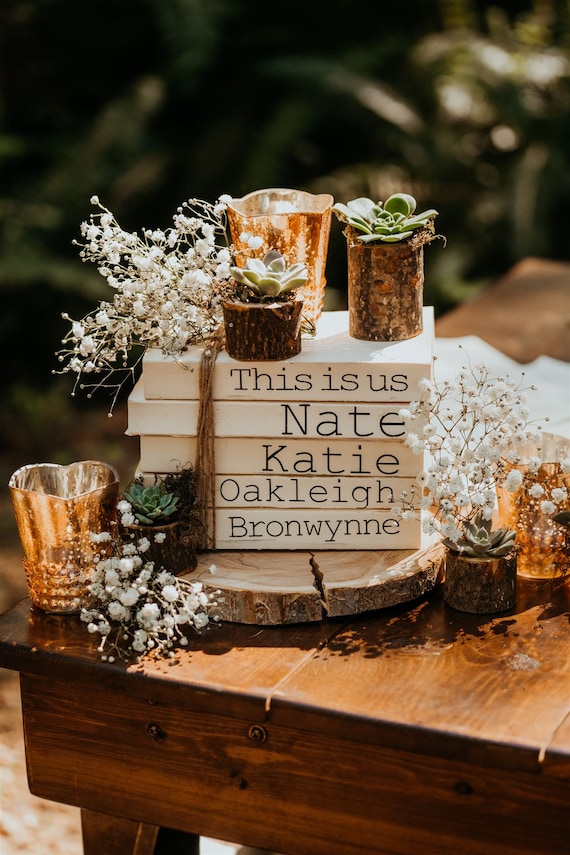The image depicts a rustic arrangement on an old, wooden table with a medium, slightly reddish hue, placed outdoors against a blurred backdrop of greenery, likely consisting of trees and bushes, under daytime lighting. Central to the setup is a slightly cracked, round wooden disk made from a tree trunk, used as a presentation plank. Stacked upon this plank are five rectangular wooden slats, resembling books, painted white and inscribed with the blue text: "This is us, Nate, Katie, Oakley, Bronwyn." 

Flanking the wooden slats are copper cups, potentially candle holders, though their exact purpose is unclear. Atop the stack of slats is another wooden piece supporting a couple of small planters made from bark, housing miniature green succulents. Surrounding the central disk are white flowers, appearing similar to cotton. The entire setup conveys a quaint, rustic charm, perfectly blending elements of wood, metal, and greenery to create an inviting outdoor scene.